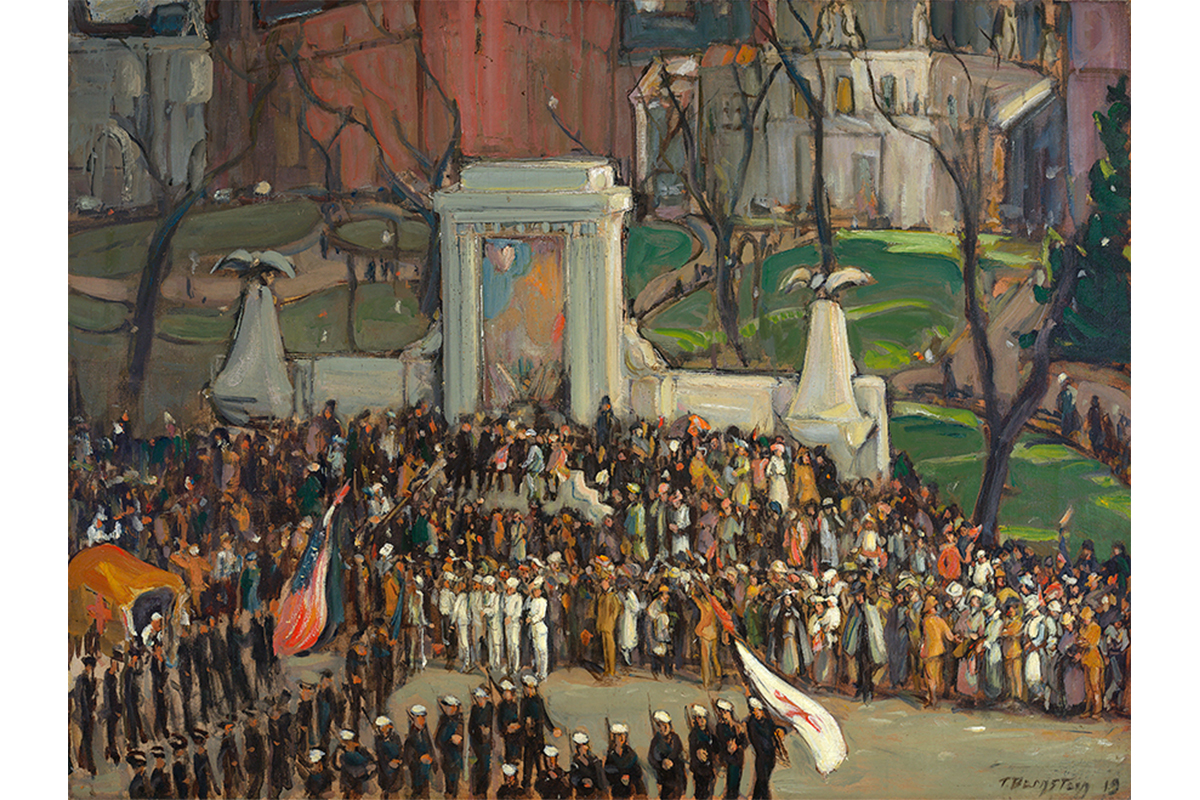The image depicts a somewhat minimalist painting or illustration of a military procession or gathering, set against an old-timey backdrop of brick buildings, some of which resemble castles in red and white hues. The foreground features a stone fence adorned with statues and an open archway. Soldiers in black uniforms with white caps stand in rows, carrying guns on their shoulders. Among them are figures in all-white military outfits, holding a white flag and an American flag. The scene includes an array of onlookers in colorful clothing, with hues of orange, blue, and white, gathered around a central area. Children are seen sitting on a ledge near a monument with pillars, which has a blue and orange painting or design on it. Various green trees painted in a watercolor style, grass, and pathways add to the scenery. In the upper right corner, buildings with solid-colored rectangles symbolizing windows shift from gray to yellow to white. At the bottom right corner, there’s a barely legible signature "TB" followed by the number 19.